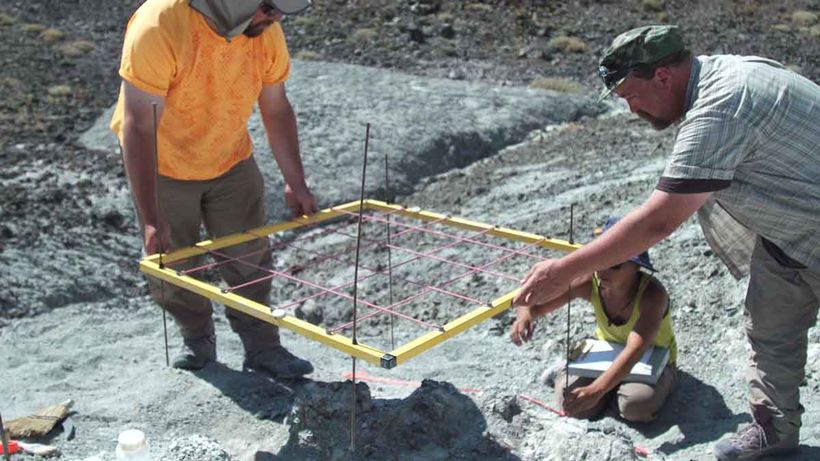In this detailed outdoor photograph, three individuals, including two adult men and one smaller person, likely a child, are engaged in what appears to be archaeological work. Central to the image is a yellow grid frame, slightly to the left, held aloft by one man on the left and another on the right. The grid, which features a yellow base and pink string, is about to be positioned on metal poles. Below the grid, another individual, wearing a yellow tank top and khaki pants, is kneeling on the ground. This person, in contrast to the adults in short sleeves and sun hats, is smaller and could be a young assistant. The adults are dressed in brightly colored clothing, with one in a bright orange short sleeve t-shirt, khaki pants, a light gray hat, and black sunglasses. The background is a mix of rocky terrain with gray volcanic rocks and brown dirt. The scene is vivid with yellows, greens, browns, oranges, and tans, reflecting the practical attire of the workers. The careful placement of the grid suggests they're preparing to excavate within its sections, typical of archaeological digs.